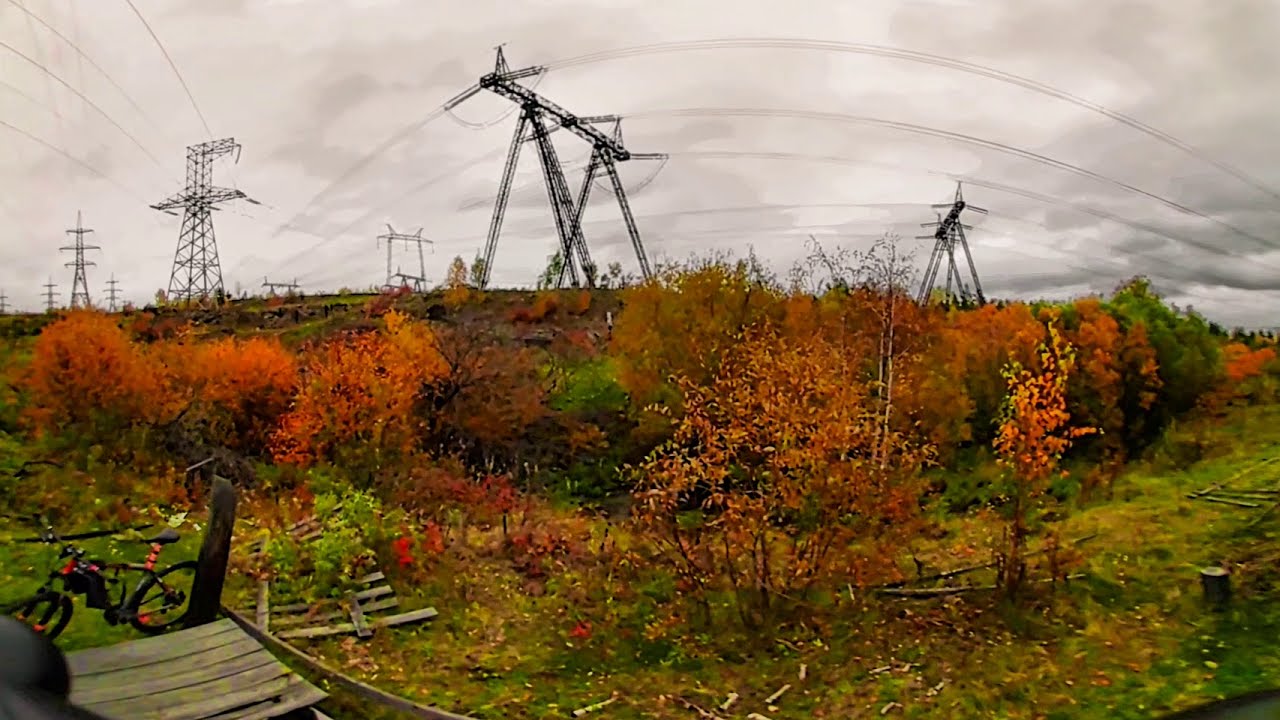This photograph captures a misty, overcast day in an industrial landscape dotted with colorful autumn foliage and expansive electrical infrastructure. The sky is a milky, grayish white, densely clouded, casting a hazy ambiance over the scene. Tall metal electrical power structures dominate the background, their colossal forms stretching into the horizon, interconnected by a web of cables. These power structures have a distinct pyramid-like shape with wide bases narrowing towards the top, and one central structure features an intricate design with triangular elements and a metal bridge.

In the foreground, the terrain is a lush green, interspersed with vibrant orange and red bushes that exhibit the rich hues of fall. The scene slopes gently, leading to a grassy area dotted with bright red vegetation and sparse green patches. To the left, a wooden walkway emerges from the lower center edge to the corner, beside which stands a black mountain bicycle with red accents. Near the bike lies a wooden picket fence, seemingly broken and laying on the ground. Despite the industrial elements, the landscape retains a natural, picturesque quality, enhanced by the seasonal colors and the subtle details of the debris and vegetation scattered across the ground.